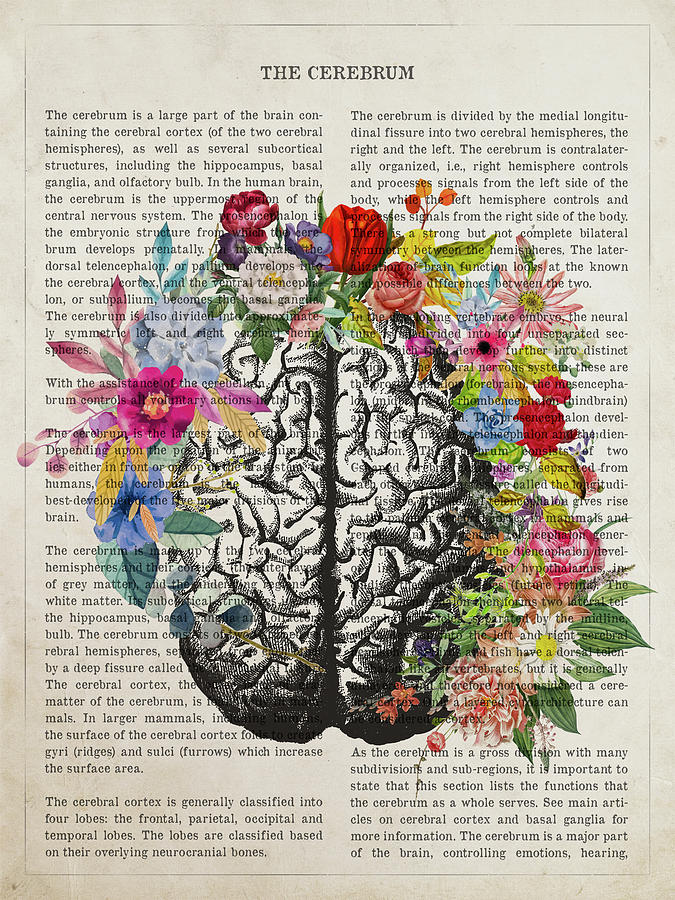The image showcases a detailed digital artwork centered around the human brain. The brain, rendered in black and white, dominates the middle of the image and is surrounded by an array of vividly colored flowers, including shades of white, pink, red, purple, light purple, and light blue. The background of the artwork is white, bordered by a black line, and filled with educational text about the cerebrum and its functions. The top middle of the image prominently reads "The Cerebrum," and the text, presented in paragraphs, elaborates on the parts and roles of the cerebrum. The combination of the monochrome brain and the multicolored flowers set against the informative text creates a visually striking and informative piece.